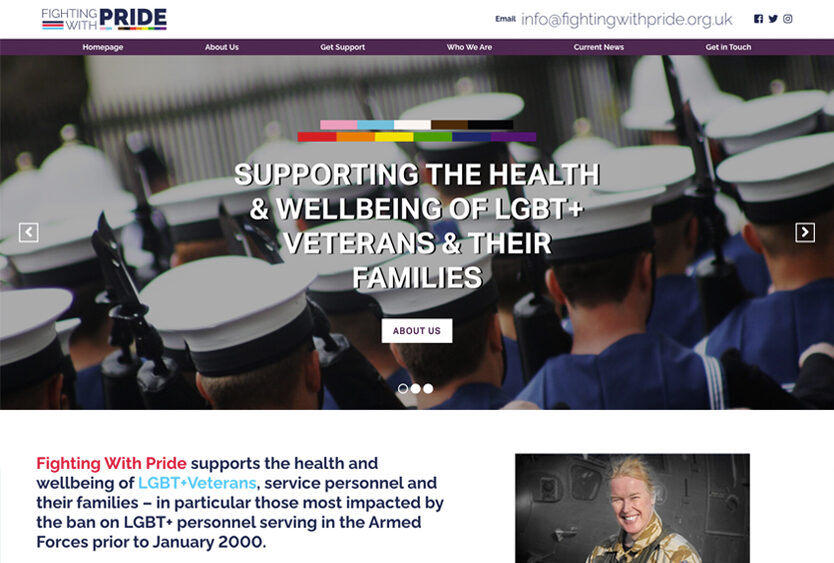The image depicts the homepage of the "Fighting With Pride" website. In the top left corner, the website’s name is prominently displayed. Below the title, there is a thin burgundy banner featuring multiple navigation tabs in white text: Homepage, About Us, Get Support, Who We Are, Current News, and Get in Touch.

Central to the image is a photograph of military personnel, identified as Navy members, wearing white hats and blue casual uniforms, which are likely not their formal dress uniforms. They hold their weapons at their left sides.

Overlaid on the photograph is a message in white lettering: "Supporting the health and well-being of LGBT+ veterans and their families." Beneath this text, a white button with purple lettering is labeled "About Us."

Further down, there is a paragraph that reads: "Fighting With Pride supports the health and well-being of LGBT+ veterans, service personnel, and their families, particularly those most impacted by the ban on LGBT+ personnel serving in the armed forces prior to January 2000."